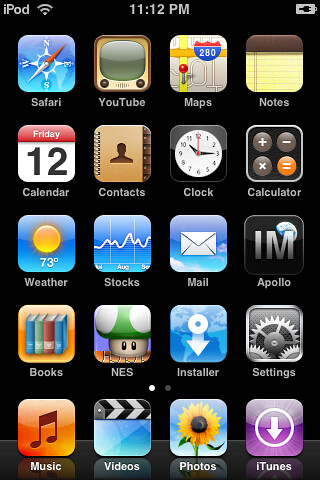The image is a detailed screenshot of an older model iPod's home screen. In the top left corner, the word "iPod" is displayed alongside a full signal strength icon. The time is shown in the center at 11:12 p.m., and on the right, there is a battery icon indicating the device is charging, marked by a small plug symbol. The screen features a black background and a grid layout of 20 app icons, arranged in four columns and five rows. 

The apps include Safari, YouTube, Maps, Notes, Calendar (displaying "Friday 12"), Contacts, Clock, Calculator, Weather (showing "73 degrees"), Stocks, Mail, Apollo, Books, NES, Installer, Settings, Music, Videos, Photos, and iTunes. Each app icon is rendered in a slightly three-dimensional style, reflecting the aesthetic of the iPod's transitional period leading up to the first iPhone release. At the bottom of the screen, the dock icons have reflective surfaces, enhancing the vintage feel of the interface. Additionally, a white navigation dot and a greyed-out dot on the bottom row suggest the presence of additional screens accessible by swiping.